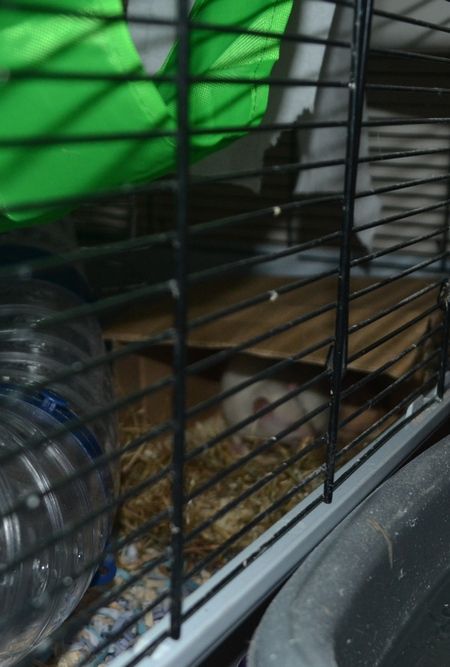This image is a detailed close-up of a pet cage, likely intended for a hamster, gerbil, or guinea pig. The cage consists of black metal bars with a light gray plastic base, and the interior is lined with sawdust bedding. Inside the cage, there are clear plastic tubes for the animal to crawl through and a piece of cardboard situated at the back, although it's somewhat hard to see. Hanging from the top of the cage is a looped piece of bright green fabric. Positioned outside the cage is a dark gray plastic bin, which appears somewhat dirty. Overlaying the entire image is a Photobucket watermark, consisting of a circular logo with concentric circles and "photobucket" written beside it in light gray text. Below the logo, a light gray horizontal band stretches across the image with semi-transparent text that reads, "Protect more of your memories for less!"